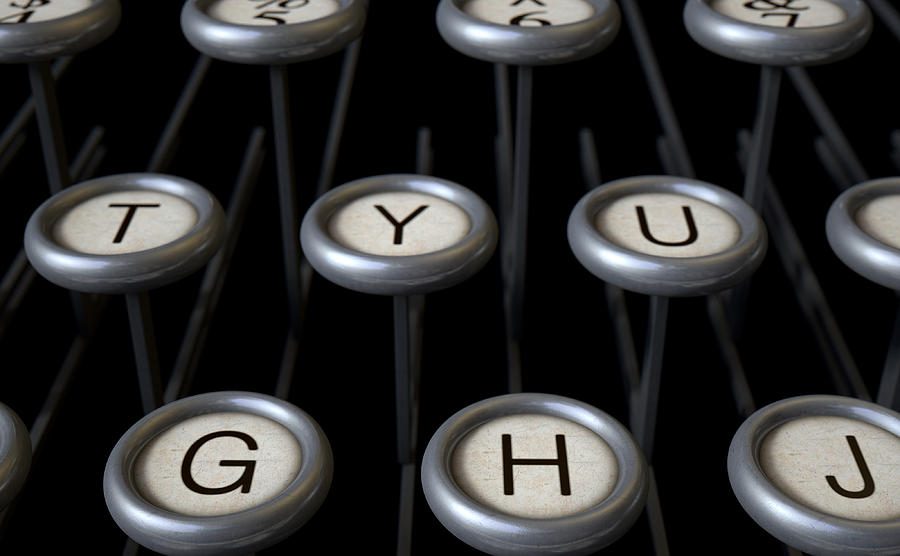The close-up image depicts the keys of an old-style typewriter, showcasing a detailed arrangement of eleven circular keys. The top row consists of numeric keys, particularly five through seven, while the middle rows display the letters T, Y, U, G, H, and J. Each key features a white background with characters rendered in a serif font, enclosed in a metallic silver ring that catches the light, giving them a shiny appearance. Beneath the keys, metal rods connect each key to the typewriter mechanism, though the intricate components remain obscured in darkness.